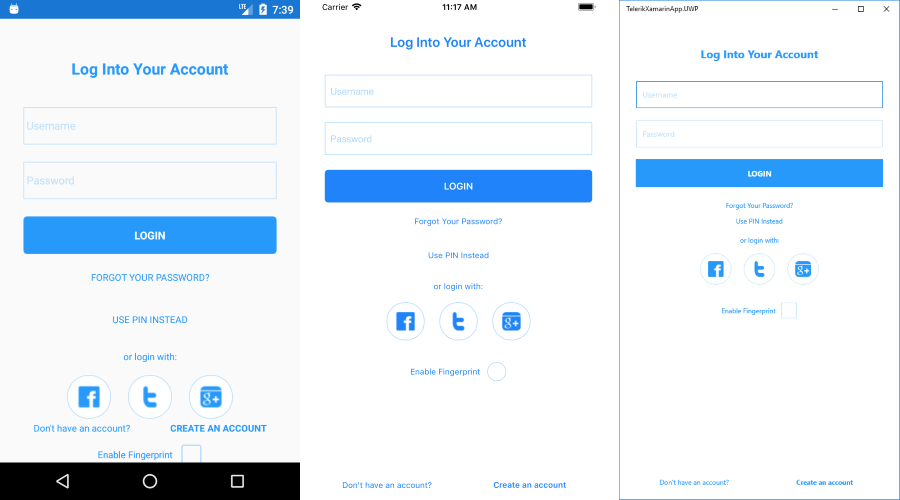The image shows a comparison of login screens across three distinct devices: an Android phone on the far left, an Apple device in the middle, and a desktop window on the right. These screens might represent A/B/C testing for layout variations or simply illustrate how the login interface appears on different platforms.

The login screen features a header stating "Log into your account." Below the header are full-width text fields for the username and password. Directly beneath these fields is a full-width login button. Under the login button are three links: "Forgot your password?", "Use PIN instead," and options for logging in via Facebook, Tumblr, or Google+.

At the bottom of the screen is an "Enable fingerprint" option, likely to utilize biometric authentication on compatible Apple and Android devices.

The design of the login screen is minimalistic, utilizing just two colors: a grayish-white background and a bright blue for the text, outlines, and buttons. This simple color scheme ensures clarity and ease of navigation for the user.